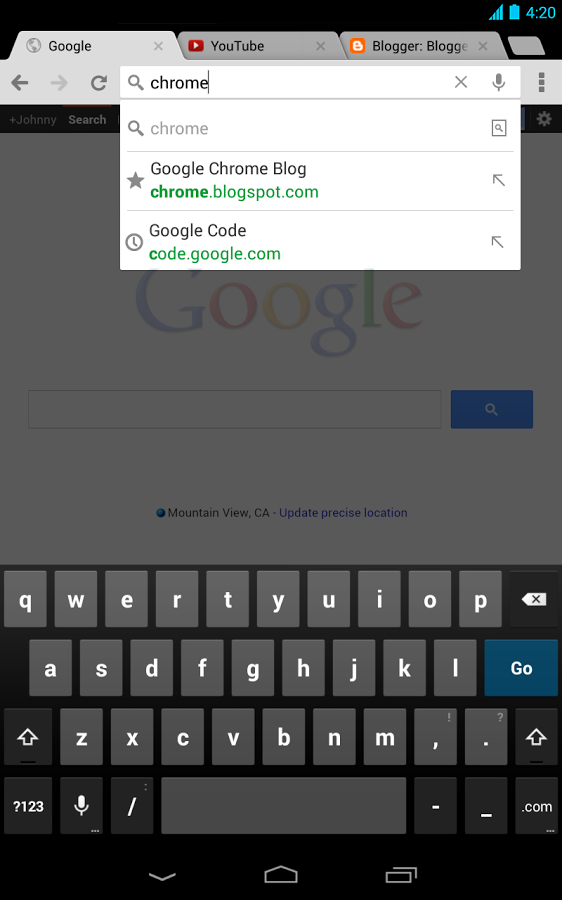This image is a screenshot taken from a smartphone. At the very top, there's a black border, and in the upper right corner, the time is displayed as 4:20 in a beautiful shade of turquoise blue. The fully charged battery icon and four bars indicating a strong wireless connection are also visible.

Beneath the status bar, the Google Chrome browser is open with three tabs labeled from left to right: Blogger, YouTube, and a Google search page. The search query entered is "Rome." A drop-down menu is shown from the URL bar, revealing that one of the search results is a Google Chrome blog at chrome.blogspot.com, marked with a gray star indicating it is bookmarked. The website URL is written in green font.

The main Google search page in the background is grayed out due to the active drop-down menu. This screenshot is indicative of being from a few years ago, as suggested by the older Google font style centered on the page rather than to the side.

At the bottom of the screen, there's a virtual QWERTY keyboard with gray keys and white letters. The "Enter" or "Go" key is in a nice shade of grayish blue. The bottom border of the screen is black, mirroring the one at the top.